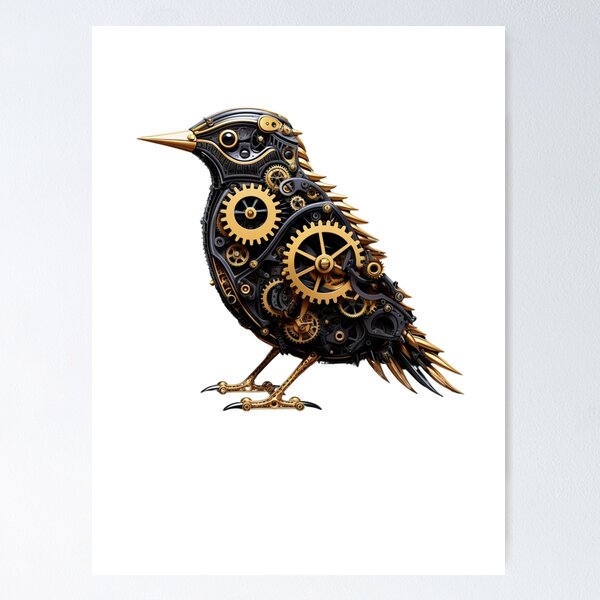This image depicts a steampunk-inspired rendering of a bird against a pristine white backdrop, with a subtle gray border enhancing the composition, reminiscent of a postcard overlay. The bird, primarily characterized by a black exterior that could be a dark blue hue, is intricately built from metallic components, prominently featuring internal gears and wheels crafted from brass or gold materials. It possesses striking gold elements including a metal beak, talons with black tips, and various feathers. Its plumage incorporates a pattern of gold spikes, especially noticeable along its tail and back, with a central black spike amidst the gold. The bird is presented in profile, gazing towards the left, showcasing its elaborate mechanical design and sophisticated aesthetic.